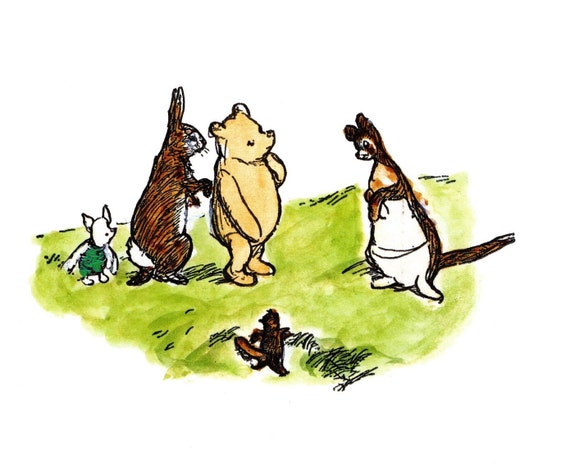In this small, boundary-less horizontal cartoon image, several beloved characters from the Winnie the Pooh series are gathered on a patch of grass, rendered as an irregular, green spot with darker green areas. At the center stands Pooh Bear, who has his hand to his mouth, appearing puzzled. Behind Pooh Bear is Rabbit, with Winnie the Pooh himself positioned as a small figure to Rabbit's side. On the right side of the image, a kangaroo is depicted, holding something in its hands, with its tail stretching out behind it and an open pouch visible. Another small figure stands facing these characters, contributing to the scene's dynamic interaction.